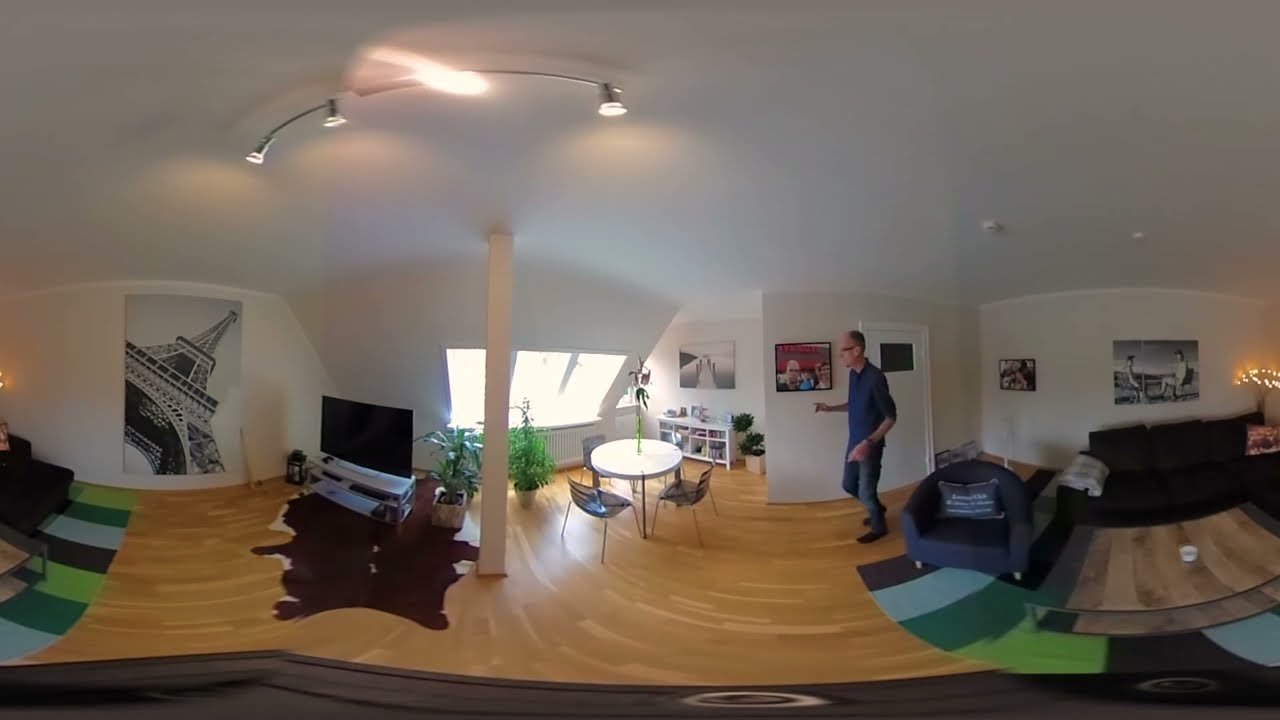This is a detailed computer-generated image of a modern apartment featuring fisheye effects on both the left and right sides. The room has white walls and a white ceiling with three lights attached in the upper left corner, casting a warm glow. The floor is made of light brown wood. Central to the composition is a Caucasian man in motion, giving an action shot appearance with his hands slightly raised. He has short brown hair, glasses, and is dressed in a navy blue shirt paired with either gray or blue pants.

The living area is furnished with a blue single-seater sofa and a black multi-seater sofa. A large, detailed picture of the Eiffel Tower adorns the left wall, alongside other artworks including images of two people sitting and a pier extending into the distance. Near the center of the room is a small round white dining table with two chairs, holding a plant.

Further details include a flat-screen TV on a stand to the left of the table, with a distinctive large bear outline rug in brown and white underneath. The room is brightened by natural sunlight streaming in from a window and possibly a skylight, creating a pleasant indoor ambiance. Several potted plants are scattered throughout, enhancing the room's aesthetic appeal.